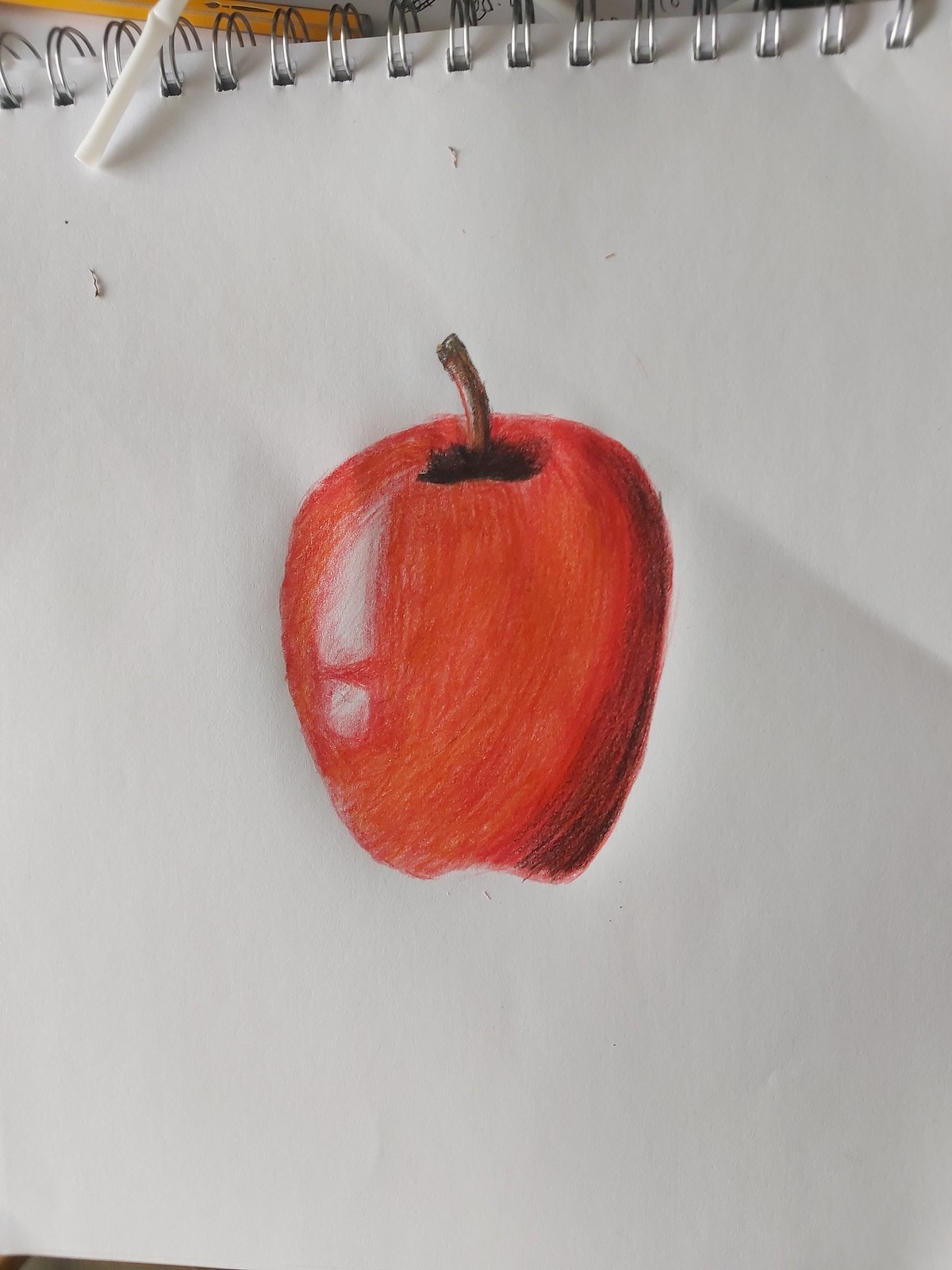"A detailed colored pencil sketch on white paper depicts a slightly undersized, red delicious apple. The artist has meticulously applied a rich, vivid red to the apple's surface and incorporated a touch of white to simulate the reflection of light, adding a realistic sheen. The apple’s brown stem emerges from a small patch of dark black at its base, enhancing the depth and contrast of the sketch. The overall effect is a lifelike representation that captures the apple's natural beauty and glossy appearance."